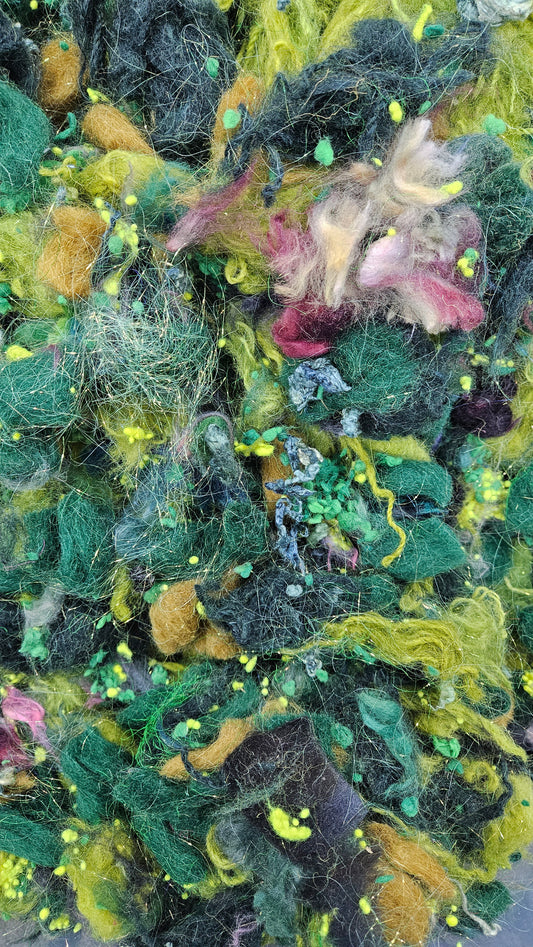The image features a close-up view of various shades and textures of fuzzy, fibrous materials intertwined and pressed together. Predominantly composed of green colors, ranging from light and mossy to dark green, the scene also includes vibrant highlights of orange, pink, white, and purple. The materials appear to be a mixture of felt scraps, frayed yarn, and fine, hair-like fibers, resembling a haphazard pile of crafting remnants. Some elements look like cotton stuffing, adding to the overall impression of a soft, yet potentially itchy, texture. The intricate, zoomed-in perspective makes the materials blend together, creating a complex, multicolored tapestry-like effect.